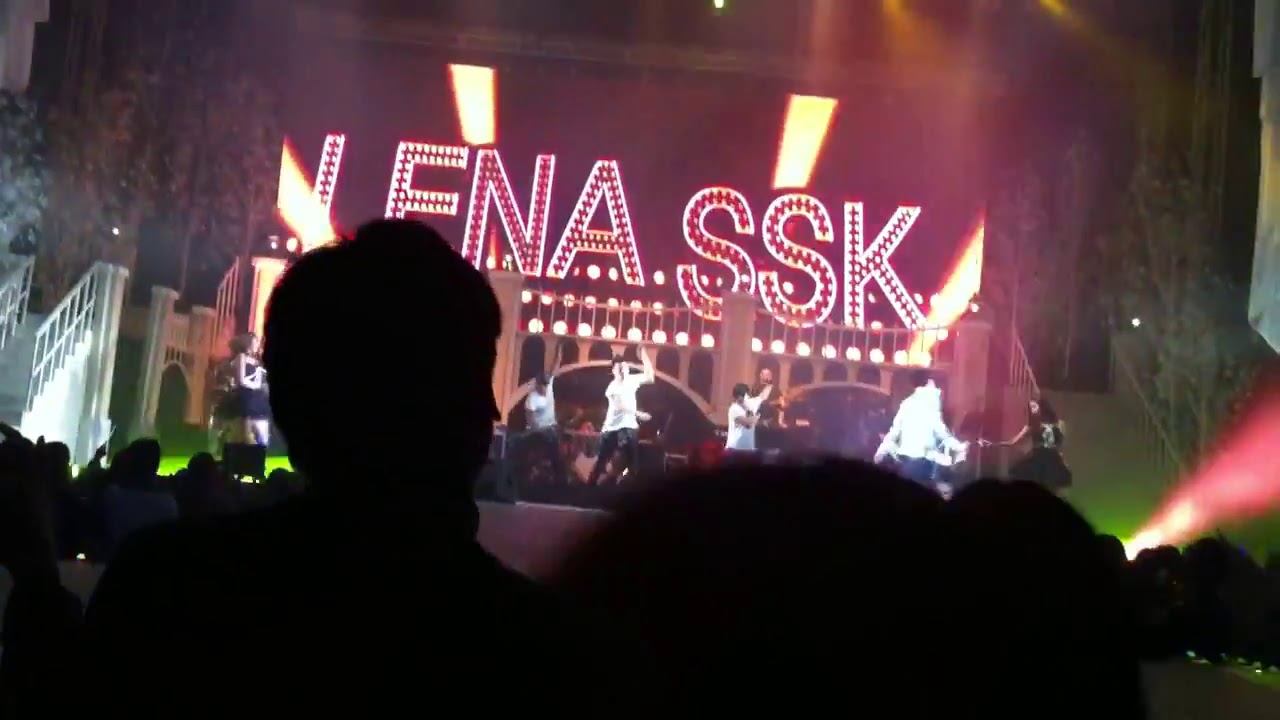This photograph captures the lively atmosphere of an outdoor musical concert taken from the middle of the audience. The crowd is seen as dark silhouettes, with the outline of heads distinctly visible on the left and right. In the foreground, the stage is brightly illuminated, featuring a vibrant mix of lime green, pink, yellow, and reddish lights. 

On stage, there are five to six performers, mostly wearing white t-shirts and black pants. They are engaged in energetic singing and dancing, with some in coordinated formations. Notably, a young girl in a black dress is either dancing or playing an instrument on the left, while on the right side, a man and a woman, possibly in a duet, are dancing with the man in white and the woman in a black dress.

Above the stage, a prominent marquee reads "LENA SSK," surrounded by white and possibly red lights, adding to the grandeur of the performance space. The stage is flanked by staircases on both the left and right edges, integrating seamlessly into the overall setup. This image vividly depicts the excitement and dynamic energy of a live musical performance, with an audience fully engrossed despite their faceless silhouettes.